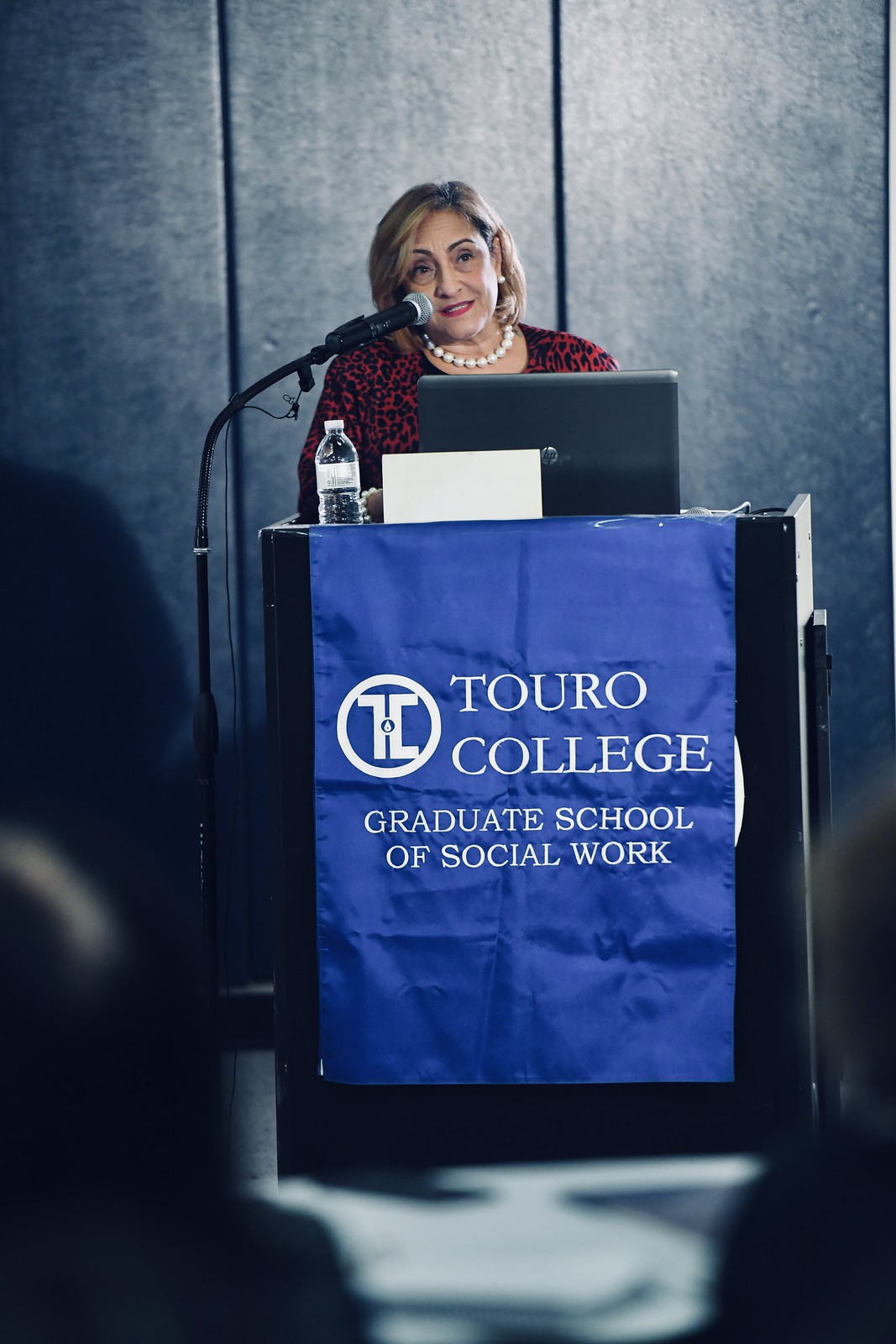In this photograph, a woman is standing behind a podium giving a speech, with a flexible microphone positioned near her mouth. She is wearing a red and black dress along with a striking white pearl necklace. Her makeup is noticeable, with red lipstick emphasizing her features. The podium in front of her holds a gray laptop and a bottle of water, and is adorned with a blue banner that reads "Touro College Graduate School of Social Work" in white text, along with the college's logo. Her blonde and brown hair falls to her shoulders, and behind her is a blueish-gray paneled wall. In the out-of-focus foreground, there are blurred images of audience members attentively listening to her speech.